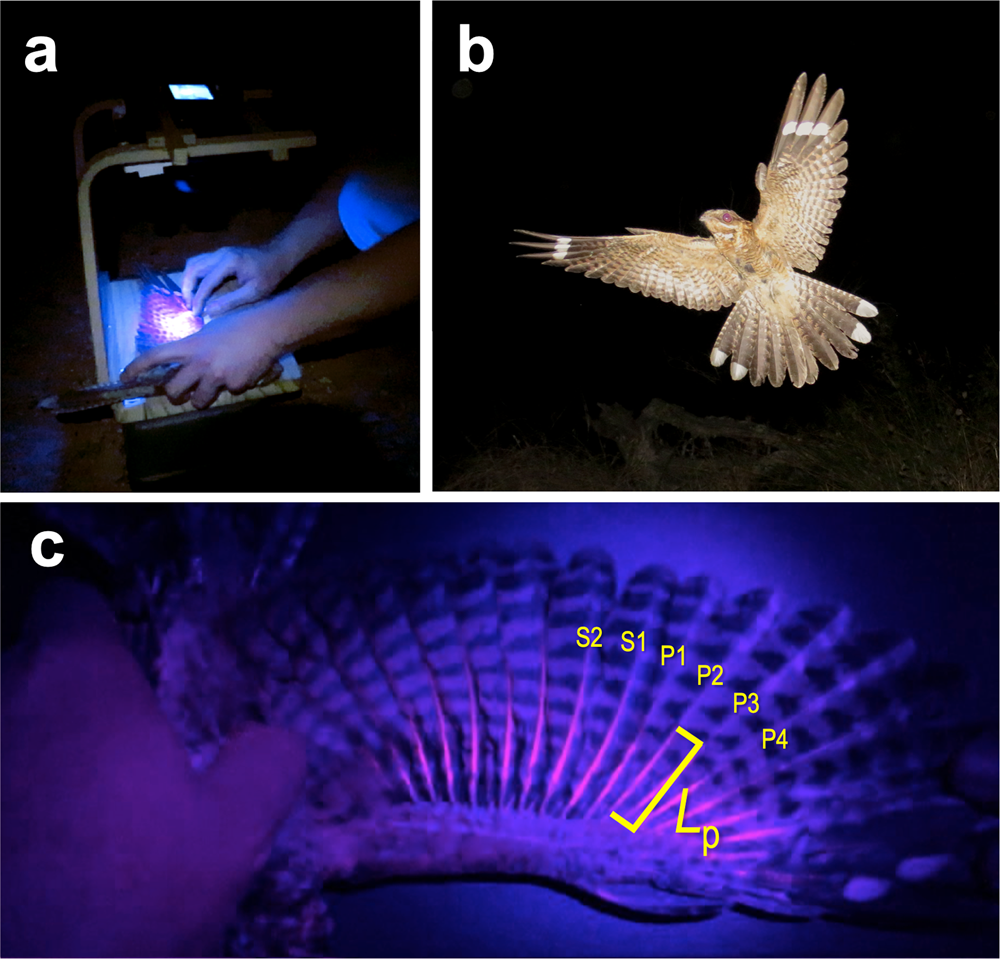The composite image features a series of three photographs distinctly labeled A, B, and C. In the top left section labeled A, we observe a man’s hands meticulously handling a bird's wing, possibly tagging it for tracking purposes. The wing is lit by a purple or pink light, and the man uses a specialized contraption to keep the bird still, ensuring a detailed examination. The scene is enveloped in darkness, highlighting the focused light on the wing.

The top right section, labeled B, captures a bird in mid-flight against a nocturnal backdrop. The bird, with its brown and cream striped feathers, is vividly lit by a camera flash. Its wings and tail feathers are outstretched, and a glint in its eyes, probably reflecting the light, gives a reddish hue.

The bottom section, labeled C, provides a close-up of the bird’s wing under the same purple light. Various parts of the wing are meticulously labeled with yellow text, including identifiers such as S2, S1, P1, P2, P3, and P4, with one section marked with a capital 'L' and a lowercase 'p'. The illuminated details suggest an in-depth study or tracking effort pertaining to the bird.